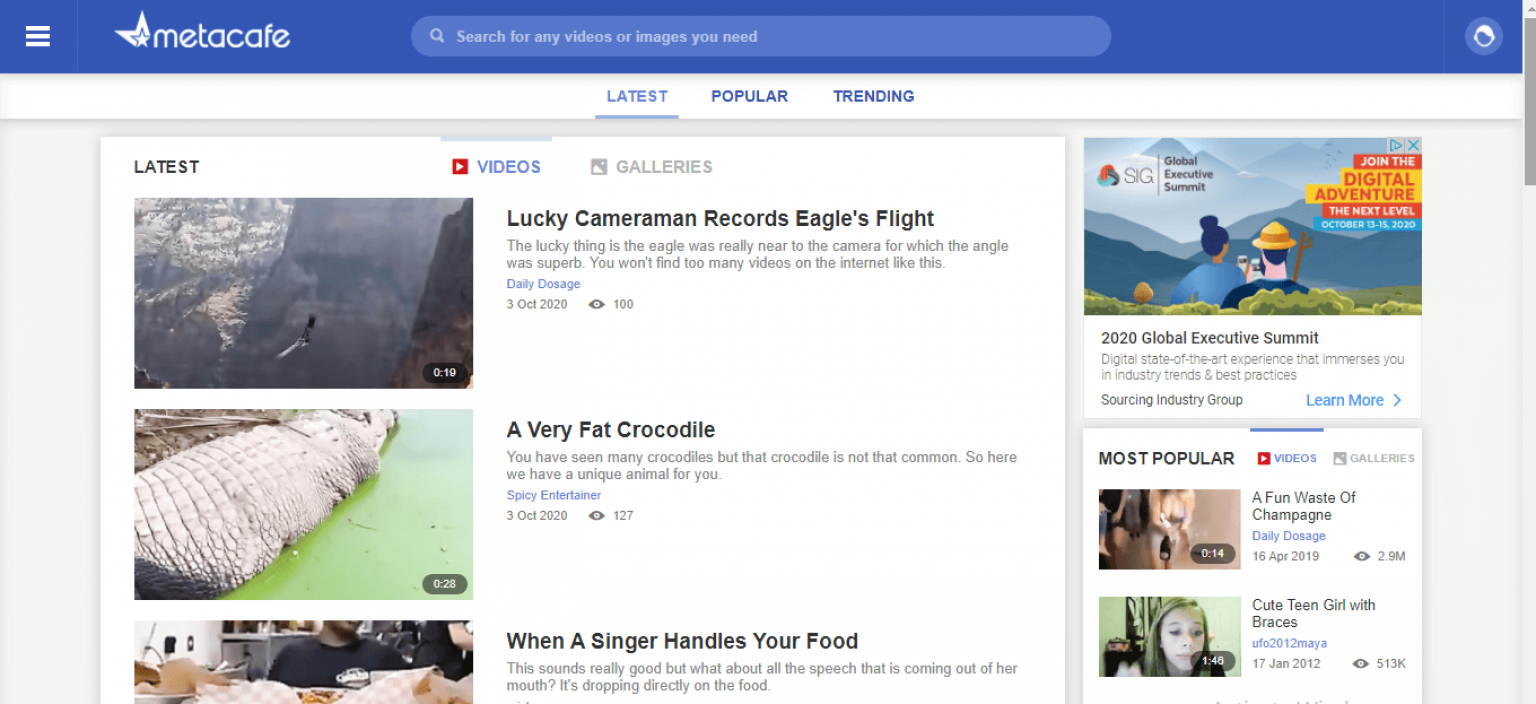The image, captured from a smart device, showcases a horizontally-oriented screenshot of the Metacafe app interface. At the top, there's a distinctive long blue rectangular bar. Positioned in the upper left-hand corner are three horizontal white lines indicating additional menu options. Beside this icon, the recognizable Metacafe logo and the word "Metacafe" are clearly visible. 

To the right of the logo, a lighter blue search bar features a magnifying glass icon and the text, "Search for any videos or images you need." Positioned in the upper right-hand corner is another small icon. Below the top bar is a white strip with a blue-highlighted and underlined label reading "Latest," indicating the currently selected category. Options to switch to "Popular" or "Trending" categories are also present.

Further down, there is another white background displaying the latest videos. Users can toggle between viewing "Videos" and "Galleries." Each video is represented with a thumbnail image, title, brief description, source, date, and the number of views. For instance, the first video listed is titled "Lucky Cameraman Records Eagle's Flight," followed by a brief description, the source, date, and view count. The subsequent videos are "A Very Fat Crocodile" and "When a Singer Handles Your Food," each accompanied by essential metadata.

On the right-hand side, there is an advertisement for the "2020 Global Executive Summit" followed by a section showcasing the "Most Popular Videos."